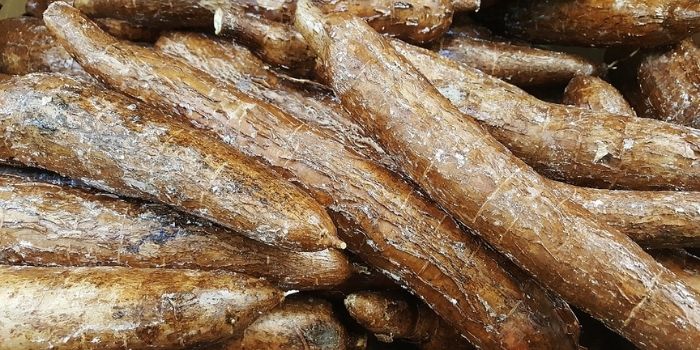The image portrays a close-up of multiple tuber-like root vegetables, resembling yams, meticulously stacked and filling the entire frame. These cylindrical objects, over ten in number, have rough, bark-like exteriors with an uneven texture suggesting some hard and jagged areas. They display various shades of brown, interspersed with marks and patches of white waxy film, and some sections appearing almost black. The tubers, positioned haphazardly atop one another, predominantly feature cut-off ends, adding to their natural, rugged appearance. Despite the photo's lack of contextual background, the detailed depiction indicates it could be taken at a farmer's market or grocery store, their phallic shapes reminiscent of cucumbers, but distinctly brown and earthy.